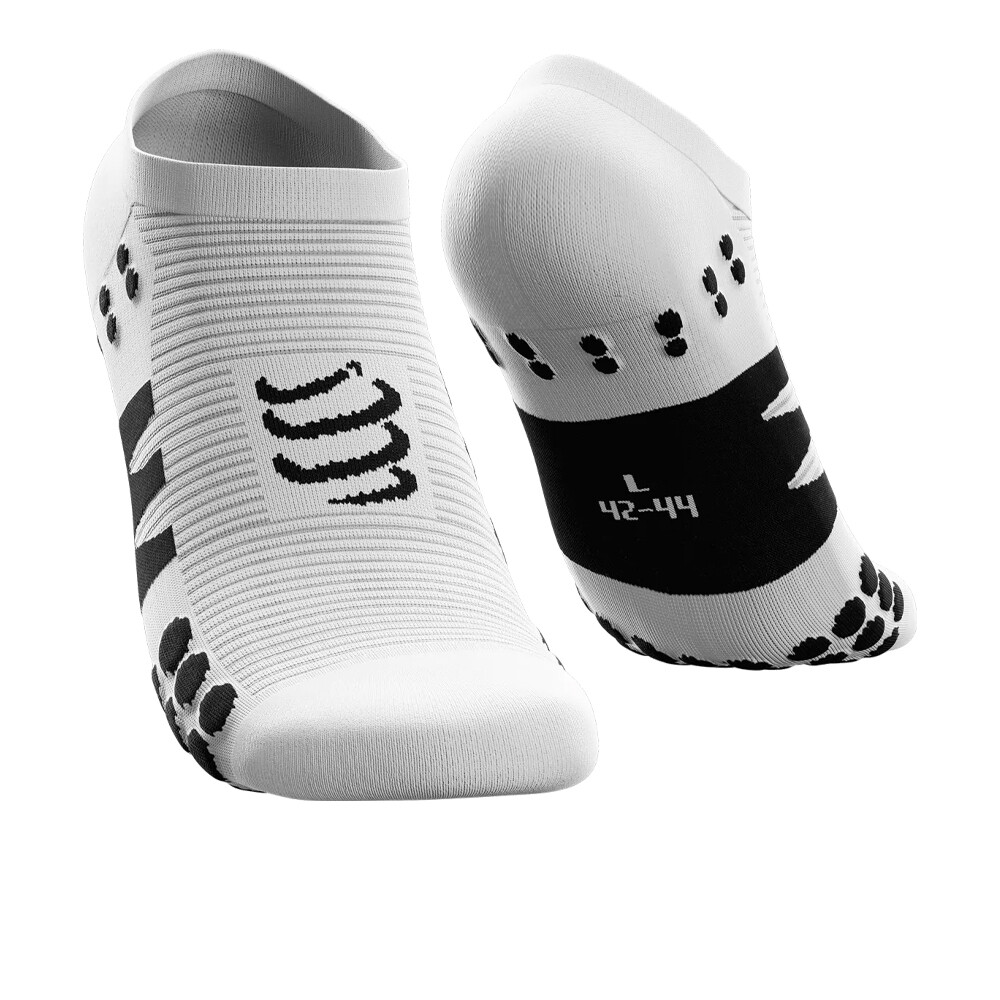This advertisement photograph showcases a pair of ankle-length, athletic-type socks designed to also function as slippers. Against a stark white background, the socks are displayed as if worn, although no feet are visible, with a potential internal frame giving them a filled-out appearance. The socks are predominantly white with intricate detailing: a series of thin, gray stripes adorns the top of the foot, while black curved swoops run vertically along the center. Circular black traction studs are sewn into the bottom fabric, providing grip similar to that found on slippers. Additional black stripes and dots accentuate the sides, and a bold black band spans the arch of the foot. On this band, the size designation "L 42-44" is prominently displayed in white lettering. The flexible fabric of these uniquely designed socks suggests a blend of comfort and functionality, merging the lines between traditional footwear and slipper comfort.